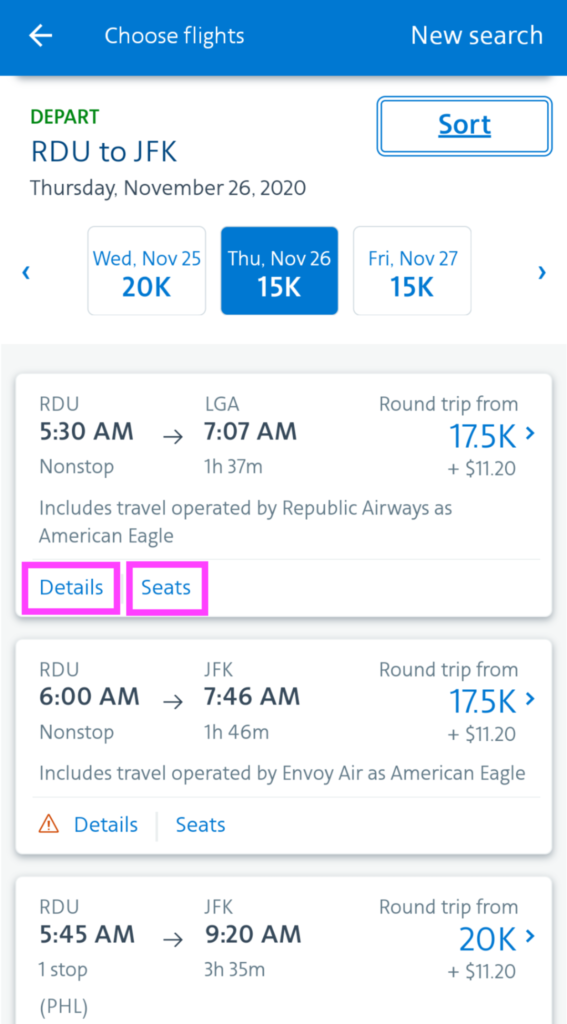The image displays a flight booking page with detailed travel options. At the top, there is an option to "Choose Flights," and a "New Search" button located at the top right corner. The page highlights a flight from RODU to GFK on Thursday, November 26, 2020. There are additional flight dates listed, including Wednesday, November 25, and Friday, November 27, with respective point costs of 20,000 and 15,000 points.

The specific flight on Thursday, November 26 departs RODU at 5:30 AM and arrives at LGA at 7:07 AM. This is a round trip costing 17,500 points plus $11.20, with a non-stop duration of 1 hour and 37 minutes. The flight is operated by Republic Airways under the American Eagle brand. Seats on this flight are highlighted in pink.

Another flight from RODU to GFK departs at 6:00 AM and arrives at 7:46 AM. This round trip also costs 17,500 points plus $11.20, with a non-stop duration of 1 hour and 46 minutes. This flight is operated by Envoy Air, also under the American Eagle brand.

The predominant colors in the image are blue and white.